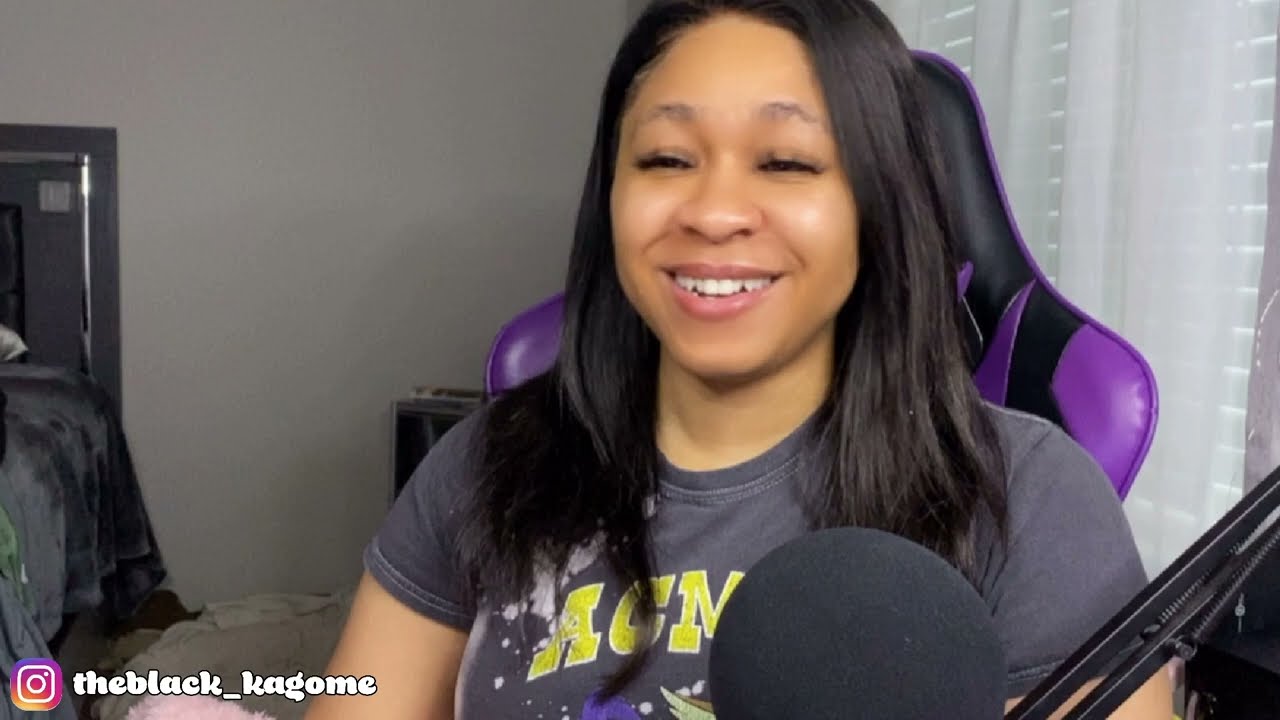This photograph captures a woman who appears to be a streamer or podcaster, presenting content from her home. She is seated in a distinctive black and purple gaming chair in what looks like her bedroom. The woman has long, black hair, neatly groomed eyebrows, and eyelashes accentuated with makeup. Her lips are pink, and she is wearing a grey half-sleeve t-shirt with a yellow "Acme" logo, hinting at a Looney Tunes design. As she speaks into a large, round, black microphone positioned in front of her, her mouth is open mid-sentence. 

The background reveals a white-themed room, including a white wall, windows with white shades, and silk-like white curtains. A portion of a black bed with a black headboard is visible to the left. In the bottom left corner of the image, the Instagram icon and the handle "TheBlack_Kagome" are displayed in white text.